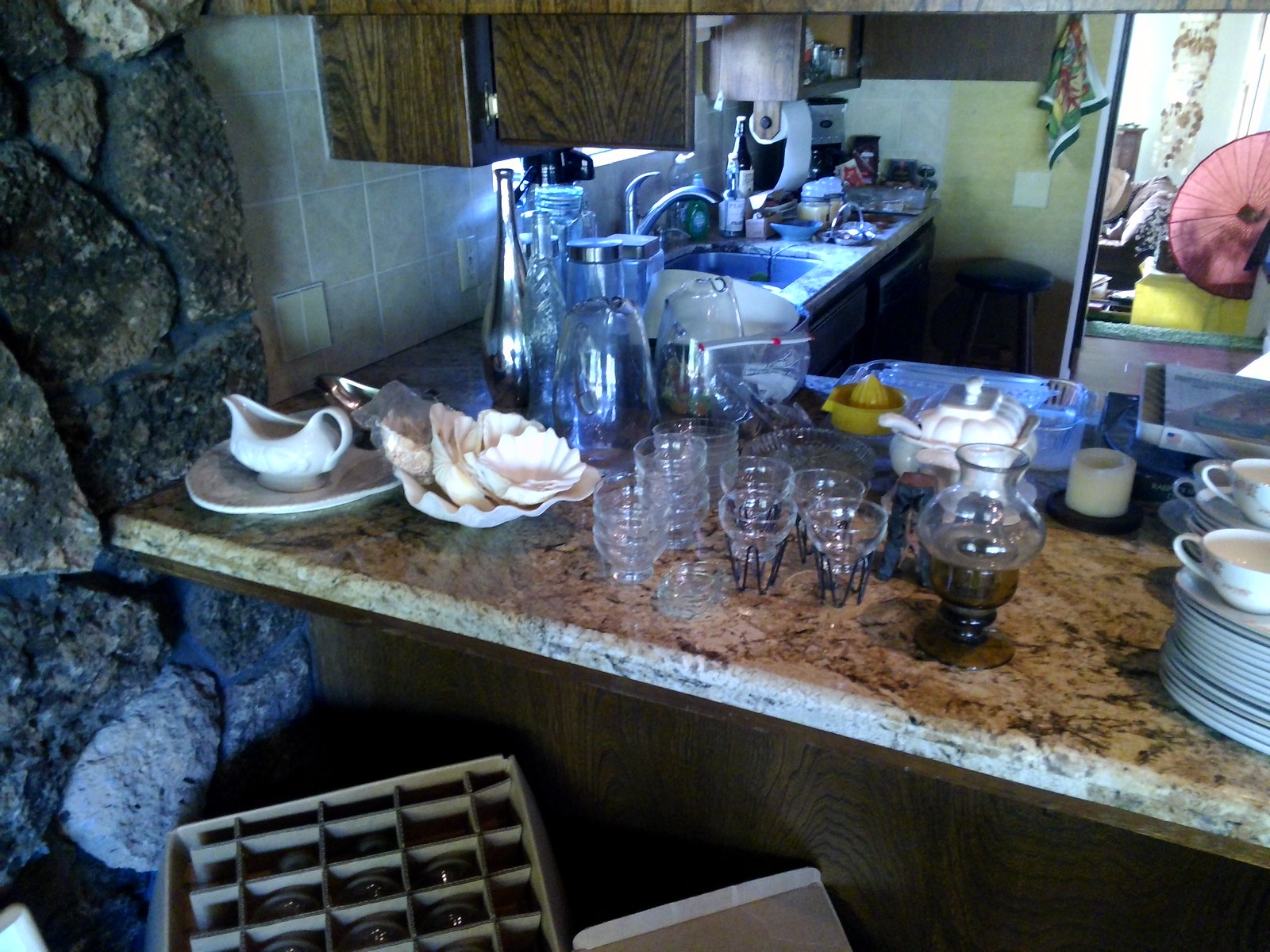The image captures a unique and rustic kitchen, meticulously prepped for hosting an event. At the heart of the scene is an L-shaped tan granite countertop laden with pristine dishware, signaling readiness for entertaining. Notable items on the counter include stacks of white serving plates, dinner plates, and smaller salad plates, alongside white china coffee cups with matching saucers. A glass casserole dish, a soup tureen, and an assortment of clear short glass bowls designed for shrimp cocktails with wire holders further embellish the surface. 

An antique-style gas kerosene lamp, a half-burned candle, and several fluted serving bowls resembling clamshells add character and charm. A serving platter with a neatly placed gravy boat stands out among the dishware. In the foreground, an open-top cardboard box holds an array of wine glasses or possibly clear bowls. 

Turning to the far side of the picture, there's a well-organized sink area accompanied by a coffee maker and a roll of paper towels, next to which a bar stool invites casual seating. Above, wood-paneled cupboards contribute to the rustic ambiance. The kitchen transitions into a backdrop dominated by a striking stone wall made of large rocks and boulders, further emphasizing the rustic theme.

Peering into the background, modern water pitchers with chrome lids, a tall opaline glass decanter, and glimpses of another room with distinctive Asian décor—including a burgundy fan and a shell macrame art piece—add layers of cultural sophistication to the scene. This richly detailed kitchen is clearly poised to delight guests with both visual and culinary appeal.